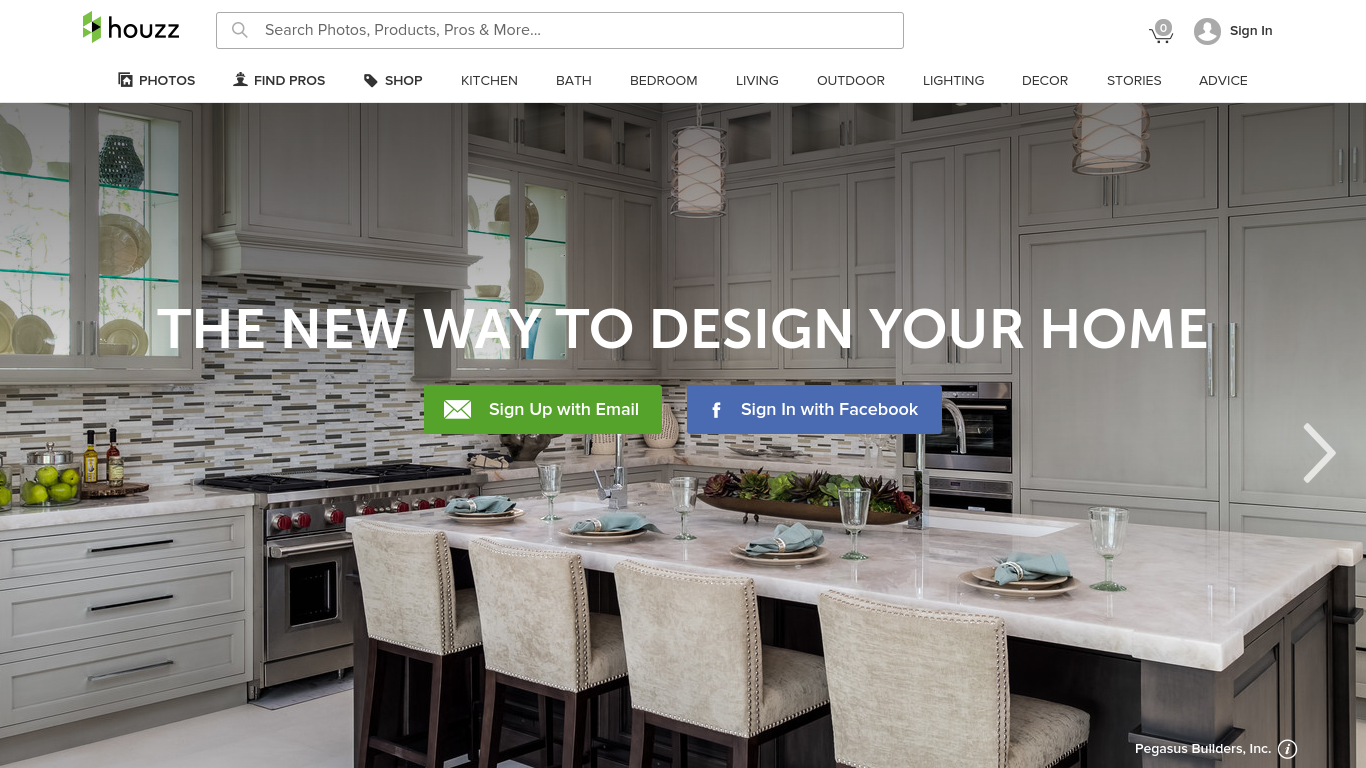The image appears to be a homepage snapshot of the Houzz website, which is a platform dedicated to home design and improvement. The website allows users to search for various products, professionals, photos, and more related to home design. The layout includes a clean, white background with vertical green squares on each side. To the left, a couple is seen browsing the site. 

On the far right, a shopping cart icon displays a quantity of 'zero', indicating that users can add items to their cart, with the count updating in real-time. Just below the primary search bar, users can find sections such as photos, pros, shop, kitchen, bath, bedroom, living, outdoor, lighting, decor, stories, and advice.

The highlighted feature in the image is a beautifully-designed kitchen showcasing a multi-colored backsplash in beige and white hues. The kitchen boasts clear white cabinets with visible dish displays, and multiple bottom cabinets. A spacious central island sits in the middle with four chairs on each side.

Central to the image, a headline reads, "The new way to design your home" in white text. Beneath this, there are two call-to-action buttons: a green "Sign up with email" button and a blue "Sign up with Facebook" button, alongside an arrow suggesting navigation to other pages or images.